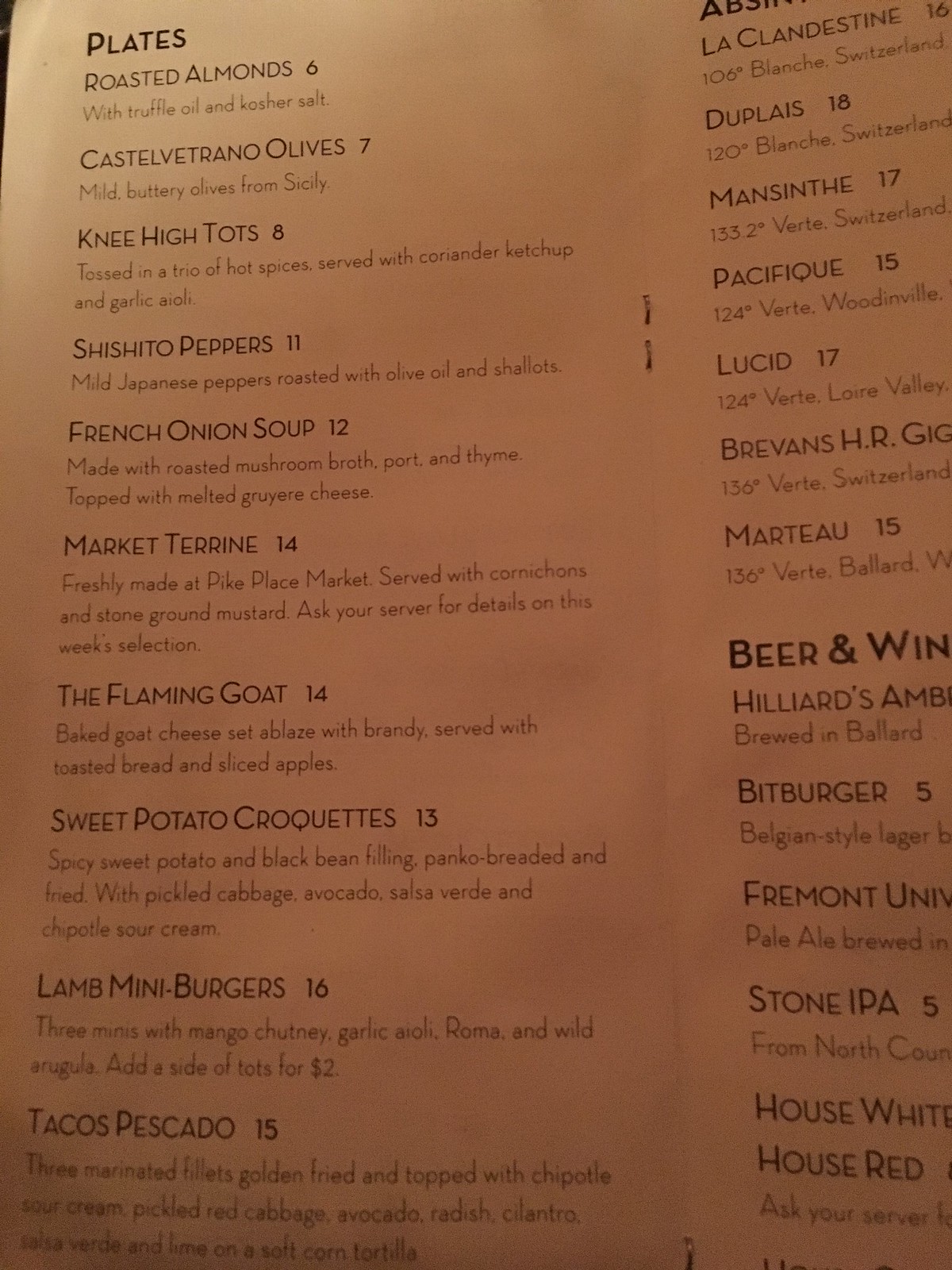A comprehensive menu, presented on a brown background, features an array of dishes and beverages. The "Plates" section offers a variety of options including: Roasted Almonds for $6, Cast of Toronto Olives for $7, Knee High Tots for $8, Shishito Peppers for $11, French Onion Soup for $12, Market Terrine for $14, The Flaming Goat for $14, Sweet Potato Croquettes for $13, Lamb Mini Burgers for $16, and Tacos Pescado for $15. 

At the top, additional intriguing selections include: Clandestine for $16, Duplies for $18, Manstente for $17, Pescafique for $15, Lucid for $17, Brevin's HR Gig, Marteau for $15. 

On the right side, a diverse selection of beers such as Hillard's Amber, Bitburger, Fremont University, and Stone IPA is listed, alongside a choice of house white and house red wines.